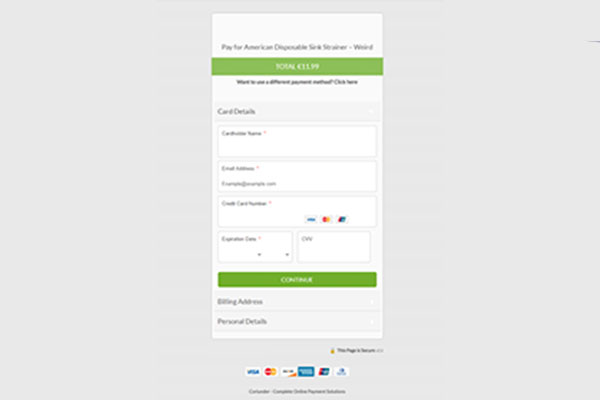The image depicts a computer screen displaying a payment form. The background of the screen is gray, and a prominent white pop-up box appears in the center, oriented vertically. At the top of the pop-up, a green strip displays a dollar amount of $11.99, preceded by a descriptive term. Below this amount, another green strip, likely a button, reads "Continue."

The form is titled "Card Details," prompting the user to enter their credit card information. Specifically, there are fields for entering the cardholder's name, the credit card number, the card's expiration date, and the CVV code found on the back of the card. Additionally, the form includes sections for the billing address and personal details, allowing space for any personal notes the user may wish to add.

At the bottom of the form, logos of accepted payment methods are displayed, including those of Discover, Visa, MasterCard, and American Express, confirming the variety of credit cards accepted for the transaction. Overall, the image provides a clear depiction of an online order page, specifically focused on the payment process.